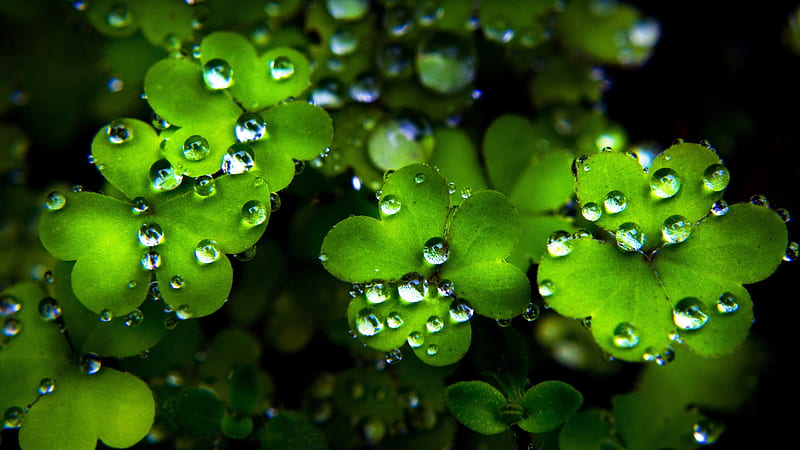The professionally taken full-color photograph, seemingly illuminated by artificial light, captures a mesmerizing outdoor scene in the dead of night. The image, horizontally rectangular, plunges into the blackness that dominates the upper right, upper left, and lower right corners, encroaching subtly into the center. The focal point, however, is a vivid cluster of four-leaf clovers. These clovers, bathed in brilliant light, appear to glow a vibrant green, starkly contrasting with the encircling darkness.

Upon closer inspection, the clovers reveal a multitude of tiny, crystal-clear water droplets, some leaves adorned with over a dozen, while others boast five or six. These droplets, reminiscent of morning dew yet heavier, catch the light, glimmering silver against the green canvas. The image's depth of field brings the foremost leaves into sharp focus, showcasing their rounded edges and intricate details, while the clovers and leaves in the background blur softly, vanishing into the dark.

Together, the glossy green clovers and their jewelled water droplets create a striking visual, illuminated against the stark, dark backdrop, potentially symbolizing good luck.